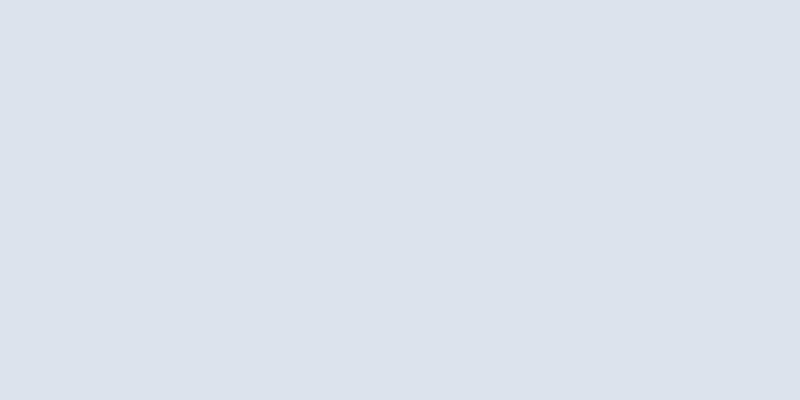The image failed to load, resulting in a gray box appearing on the screen. The gray box features a subtle gradient, transitioning from a darker gray in the top left-hand corner to a lighter gray in the bottom right-hand corner. Despite the slight variation in tonality, the screen remains largely monochromatic and empty, reminiscent of vintage mood screens designed to subtly shift colors over time.